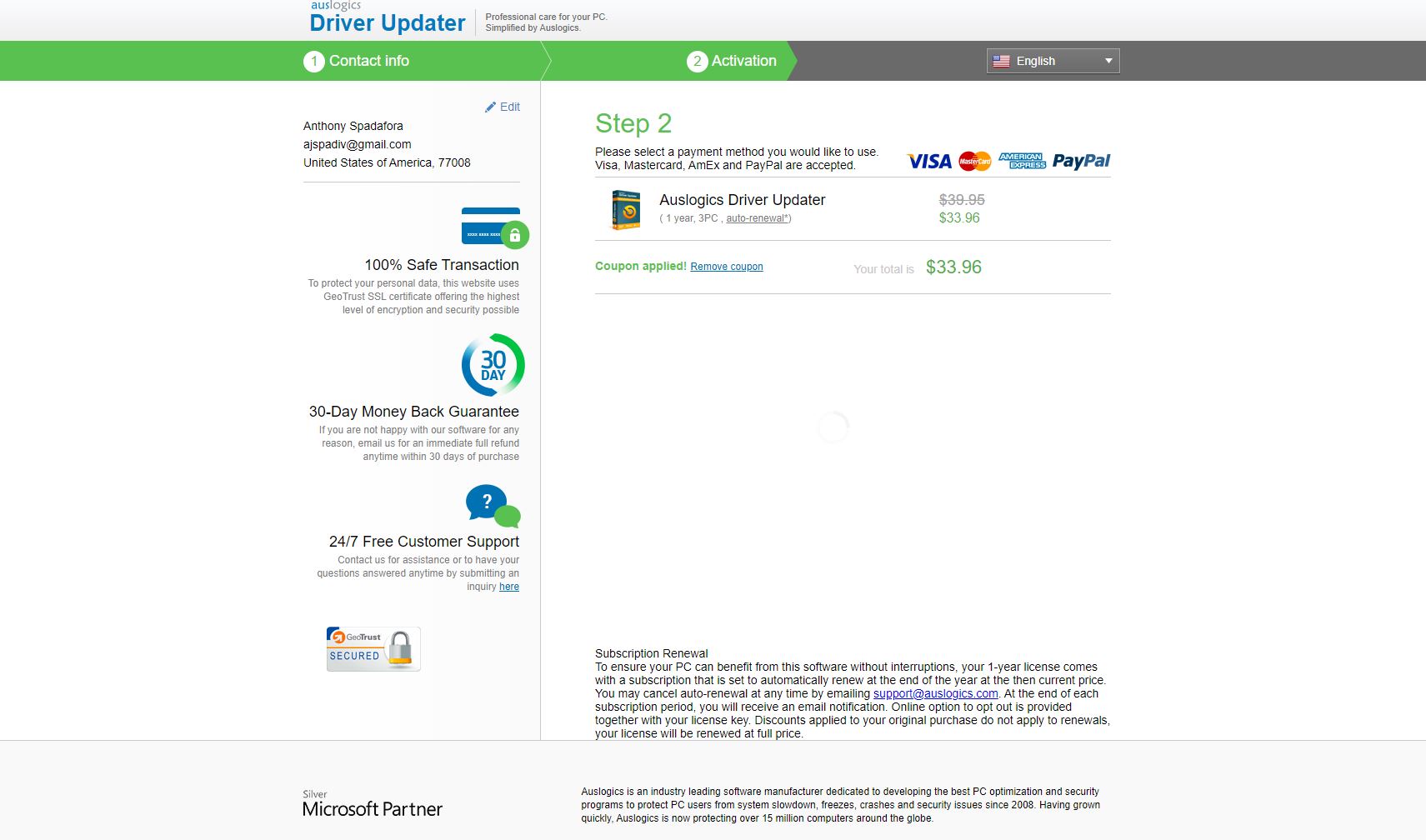This image is a screenshot from a web page for Auslogics Driver Updater. At the very top, the header is split into two colors: green on the left and gray on the right, with the text "Driver Update" displayed prominently in blue font. To the left in the green section, the header includes "Contact Info" written in white font, and towards the center in the gray section, "Activation" is also written in white font. They are labeled respectively as numbers 1 and 2.

Directly beneath the "Driver Update" header, the name of the purchaser and their email address are displayed, indicating a personalized transaction. Below this, several assurances are listed: 
1. "100% Safe Transaction"
2. "30-Day Money Back Guarantee"
3. "24/7 Free Customer Support"

To the right, under "Step 2," the text instructs the user to "Please Select a Payment Method." Four payment method icons are displayed, indicating that Visa, MasterCard, American Express, and PayPal are accepted. The cost of the Auslogics Driver Updater is clearly marked as $33.96.